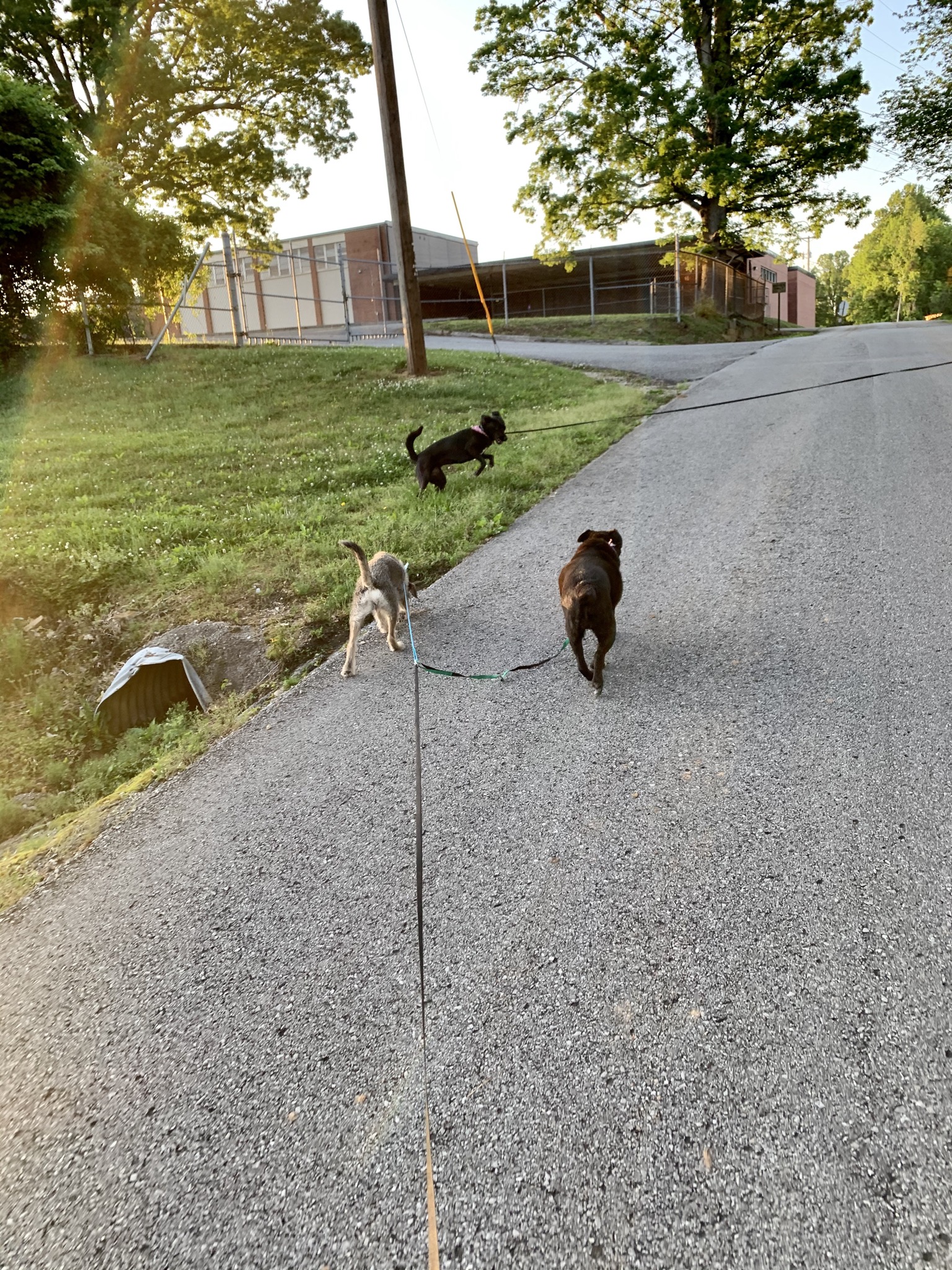In the image, a person is walking three dogs on a grey, paved road. Two of the dogs are leashed together using a long brown leash, while the third dog is ahead on a separate leash. To the left and center of the scene, there's a stretch of greenery and trees, offering a touch of nature. Just slightly to the left, where the road intersects another section alongside a chain-link fence, stands a brown pole. In the grassy area where the dogs are walking, there's a small metal drainage hole. Further to the left is a brown brick building with grey side panels, resembling either a warehouse or a school, and it features a secondary partition close to the road. The sky is clear with a blue hue, devoid of clouds and direct sunlight. In the distant background, the road stretches towards another cluster of trees illuminated by sunlight.